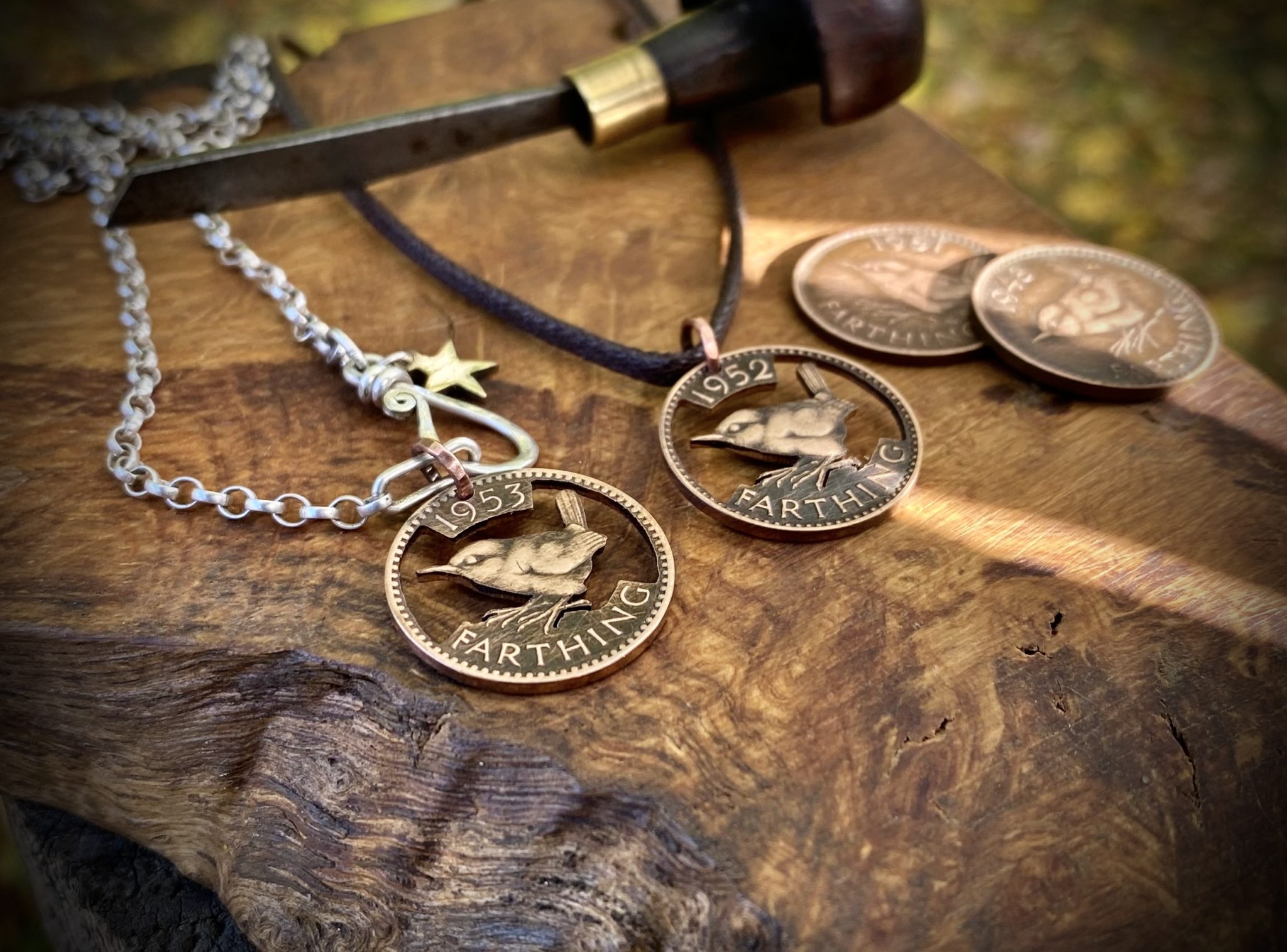This photograph captures the intricate process of crafting homemade jewelry from antique coins, presented against a rustic, multi-toned brown wooden slab. Central to the image are four brass-like Farthing coins, two of which retain their original form, while the other two showcase detailed craftsmanship. The modified coins, dated 1952 and 1953, feature a finely embossed bird facing left, with the background meticulously punched out to create an open design.

On the left, the 1953 Farthing coin is suspended from a long, silver chain adorned with a lobster clasp and a dangling star charm. The 1952 coin, on the right, is strung onto a black cord, offering a contrasting yet complementary look. Both coins retain the distinctive text "Farthing" along their lower edge. The scene is further animated by a specialized punch tool, characterized by a large metal blade, a wooden handle with gold trim, casually laid across the chains, hinting at the artisan's active role in the creation.

This array of jewelry items and tools is illuminated by sunbeams that filter across the wooden surface, set against a softly blurred green background, suggesting the photograph was taken outdoors. The careful arrangement of the elements evokes a sense of meticulous craftsmanship and the timeless allure of transforming historical artifacts into wearable art.